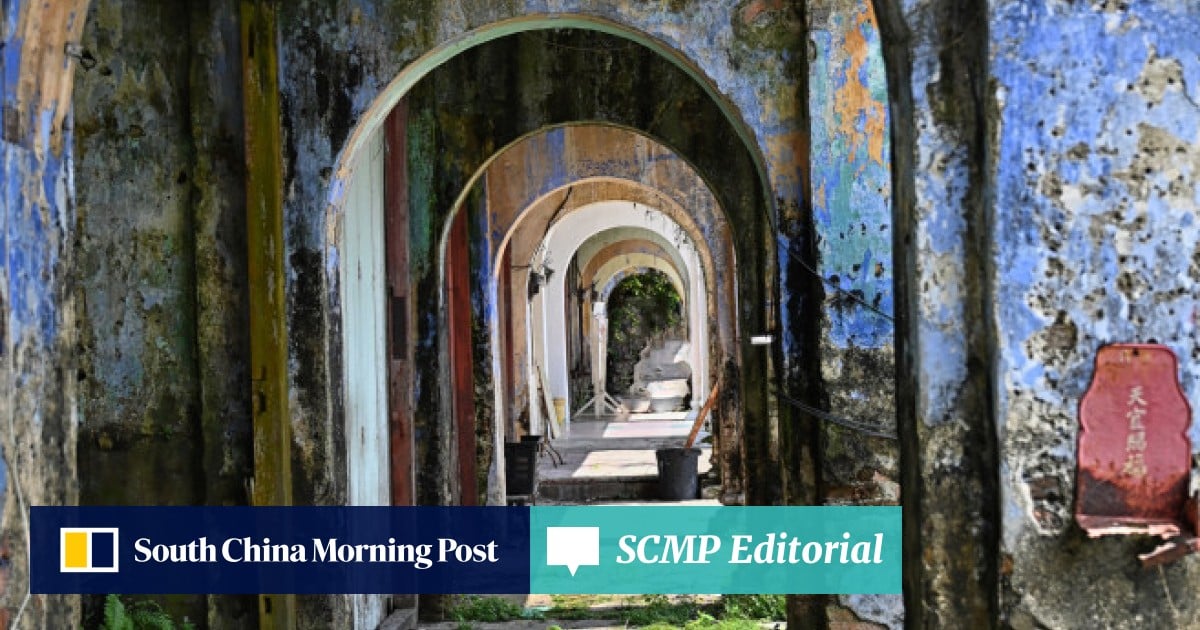This is a color photo prominently featuring a dilapidated arched walkway within a deteriorating building. The hallway is lined with six oval-shaped doorways and extends in an ongoing sequence, creating a sense of depth. The walls of the corridor are severely chipped and flaking, exposing layers of faded paint in shades of blue, yellow, red, brown, and white. Among the decay and faded hues, there are orange accents and patches of rust, emphasizing the structure’s age and neglect. A prominent feature on the right side of the wall is a rectangular red plaque adorned with Chinese lettering. At the bottom of the image, text reads "South China Morning Post SCMP Editorial," with the left text box being blue and the right light green. Two symbols accompany the text box. The image quality is fairly adequate, capturing the intricate details of degradation and vivid color contrasts.